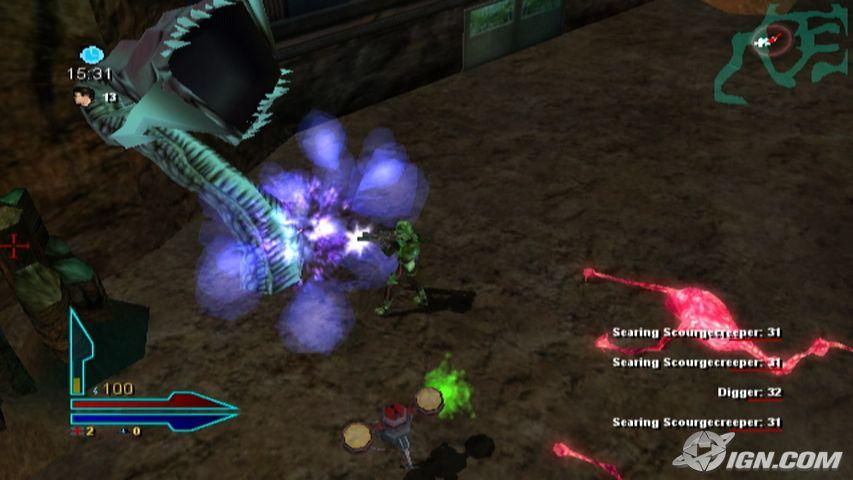This image is a screenshot from a video game, prominently featuring a vivid scene captured in mid-action. A large, menacing blue monster, with its neck protruding from the ground and a gaping square mouth lined with sharp, pointy teeth, dominates the left side of the frame. Blue plumes of smoke surround the creature as it faces off against a green-clad character shooting at it, indicating an intense battle. In the lower left corner of the image, a vibrant red and blue arrow symbol is displayed with the number 100 above it. Adding to the chaotic scene, a sizeable pink bird lays dead on its side in the same corner. The bottom right corner features a circular logo surrounded by a ring, marked with the text "IGN.com," indicating the source of the image. A detailed teal-colored map in the top right corner outlines various pathways, providing strategic information for the gameplay.